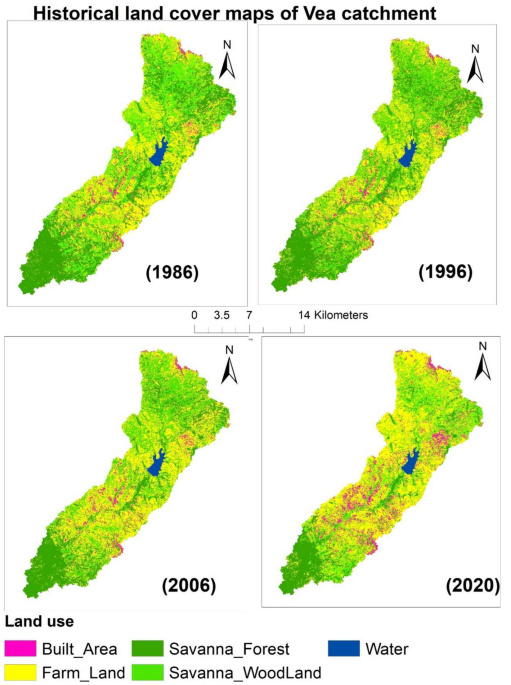The image presents a series of four historical land cover maps of the Via Catchment region, each denoting different years: 1986, 1996, 2006, and 2020. These maps are organized in a 2x2 grid with 1986 and 1996 on the top row, and 2006 and 2020 on the bottom row, with each map's year labeled in black text at the bottom right corner. Above these maps, in black lettering, is the title "Historical Land Cover Maps of Via Catchment." Accompanying the maps is a legend labeled "Land Use," which clarifies the meaning of various colors used in the maps: pink for built area, dark green for savanna forest, light green for savanna woodland, blue for water, and yellow for farmland. The maps utilize these color codes to demarcate changes in land use over time, highlighting an increase in built areas and farmland.